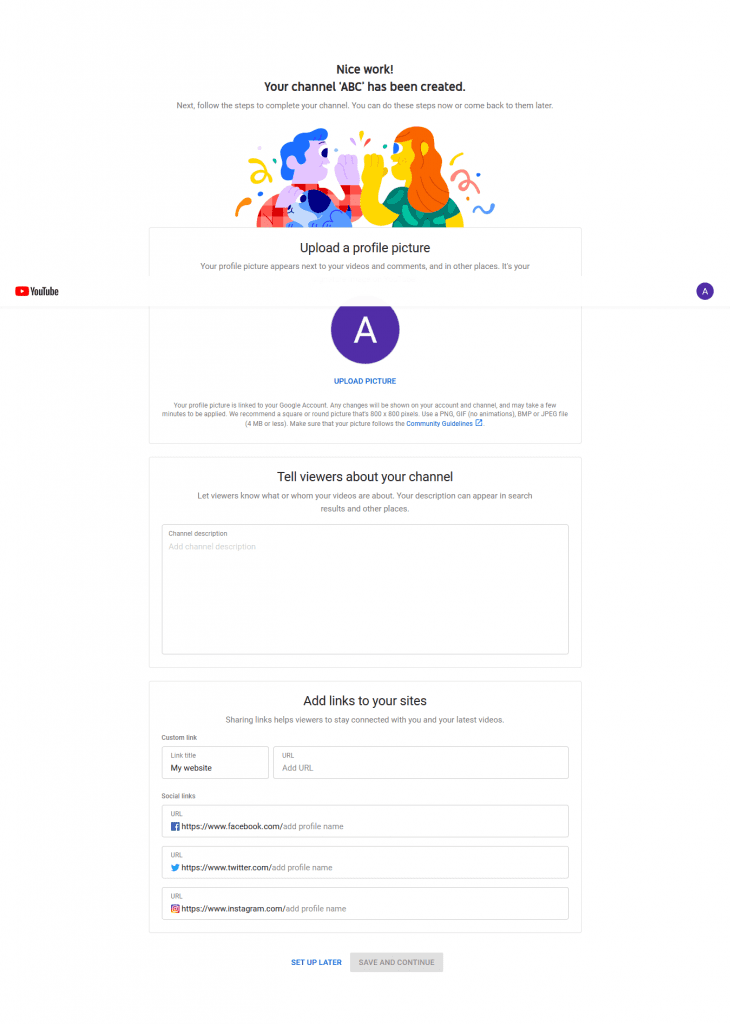In the image, there is a screenshot of a website creation tool specifically for creating a channel named "ABC". At the top of the page, it congratulates the user with the message, "Nice work! Your channel 'ABC' has been created." Below this banner, there is a cheerful clipart illustration of two characters high-fiving each other, adding a sense of accomplishment and celebration.

Further down, there's a section dedicated to adding a profile picture. Within this segment, a purple circle with the letter "A" inside is prominently displayed, indicating that the default profile picture is currently a placeholder. Beneath this, the button labeled "Upload Picture" invites users to personalize the channel with their own image.

A small, unreadable paragraph is also present, presumably containing instructions or additional information. Next, there is a prompt titled "Tell viewers about your channel" accompanied by a large text box designated for adding a descriptive summary about the channel's content and purpose.

Following this is a section labeled "Add links to your sites" which includes two input fields where users can insert URLs to their social media platforms. Visual cues suggest the links could lead to Instagram, Twitter, and Facebook, enabling channel creators to share their social media presence with viewers.